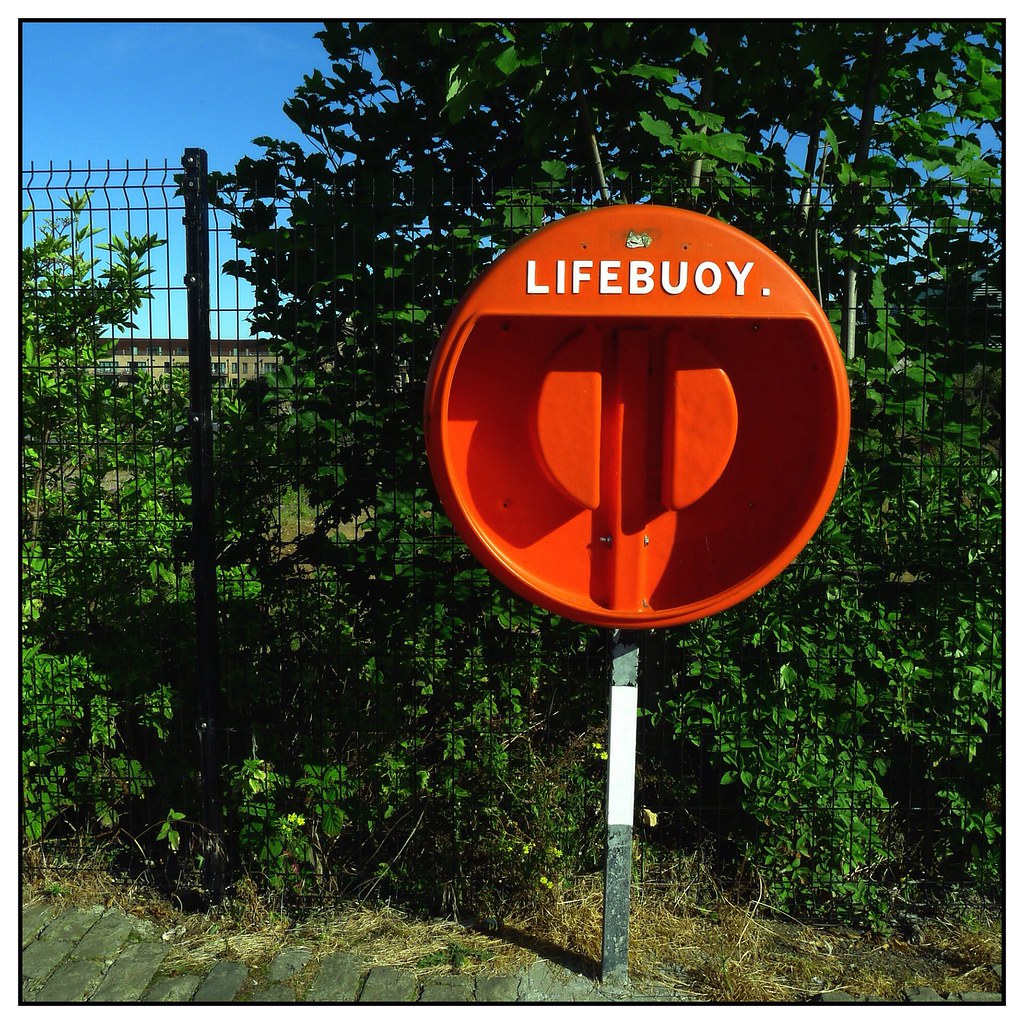This color vertical photograph depicts a vacant housing unit for a flotation ring, prominently featuring an open, circular, red casing with "Lifebuoy" inscribed in large, white capital letters. The housing, meant to contain both a flotation ring and accompanying rope, currently stands empty. It is mounted on a square, dark and white painted post, set against an older wire fence partly shrouded by tall green shrubs and a high-growing, almost weed-like, tree. Below the fencing and greenery, there are weathered brick-shaped pavers and patches of untended grass. A bright blue sky spans the top of the image, its view partially obstructed by the lush foliage. A small, green, mostly scratched-off label resides above the "Lifebuoy" inscription, while a building can be faintly seen on the left-hand side, partially hidden by the abundant plant life. The entire scene suggests a neglected yet essential safety installation, likely positioned near a beach or boardwalk setting.